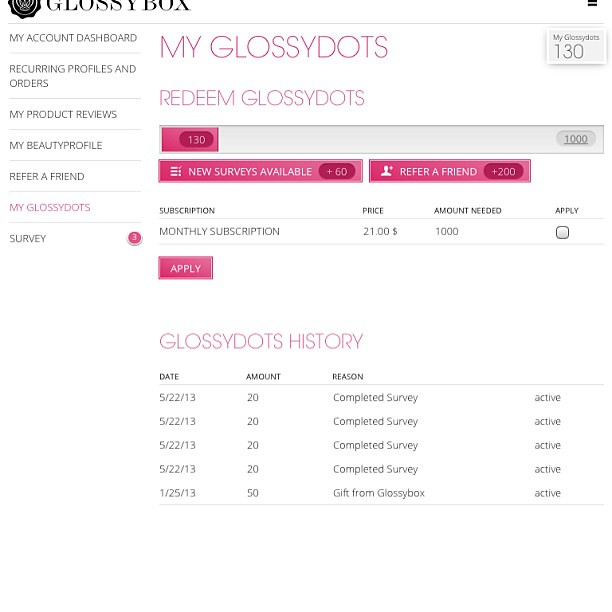This image is a screenshot of the Glossybox website, specifically the user's account dashboard. In the upper left corner, the Glossybox logo and name are displayed in black text on a white background. Below this, there are several sections listed in black lettering: My Account Dashboard, Recurring Profiles and Orders, My Product Reviews, My Beauty Profile, Refer a Friend, My Glossy Dots, and Survey.

To the right, in bold pink text, it says "My Glossy Dots" and "Redeem Glossy Dots." A pink bar indicates that 130 Glossy Dots are available, but 1000 are needed to redeem them. It also notes that a new survey is available, showing "+60," "Refer a Friend +200," and indicating that the monthly subscription price is $21. Additionally, it mentions that 1000 Glossy Dots are required.

Lower down, the Glossy Dots History is listed with details of points accumulated: $5.20 and $22.13, with four surveys completed at 20 points each on dates May 13th, May 22nd, and a gift of 50 points from Glossybox on January 25, 2013. This section also features pink and white text and includes an "Apply" button. The overall layout provides a detailed scorecard and tracking information for the user's activity and Glossy Dots accumulation on Glossybox.